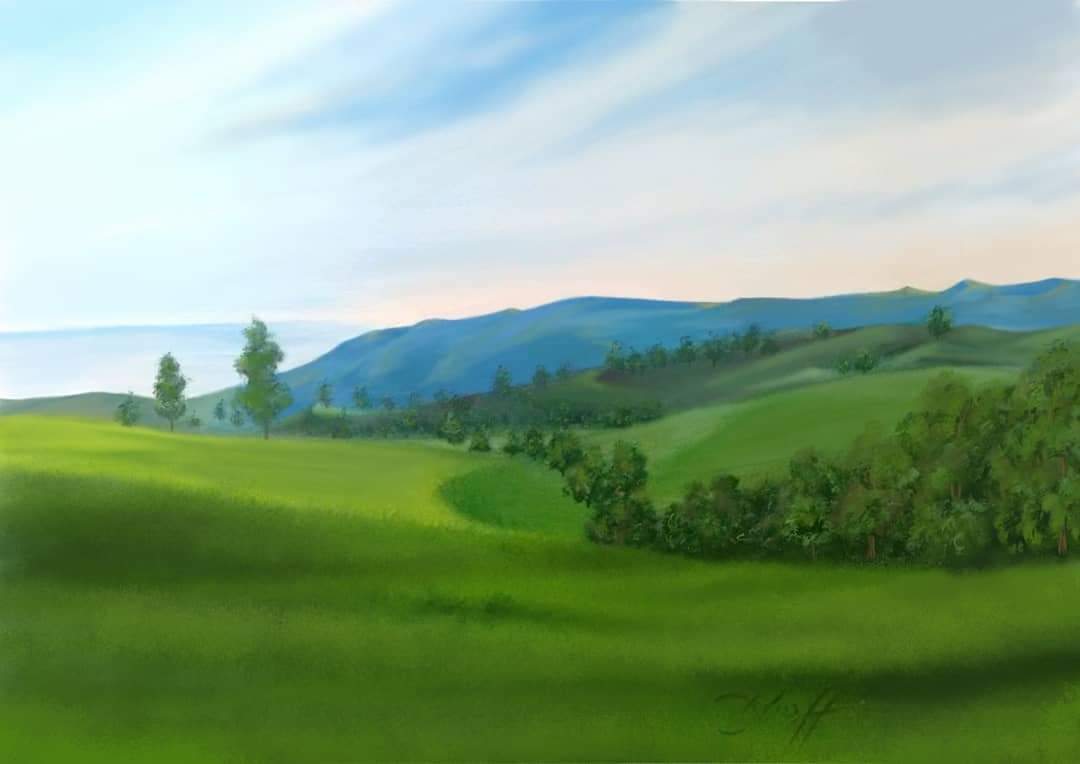A beautifully detailed landscape artwork captures a serene scene under a predominantly cloudy, yet light, blue sky. The horizon extends into the far distance on the left side with an indistinct stretch of land. Central and right in the background, gentle hills rendered in bluish-green hues add depth and tranquility to the vista. The foreground is vibrant with lush, bright green hills dotted with orderly rows of trees, punctuated by a few taller, solitary trees, enhancing the natural beauty and pastoral charm of the scenery.